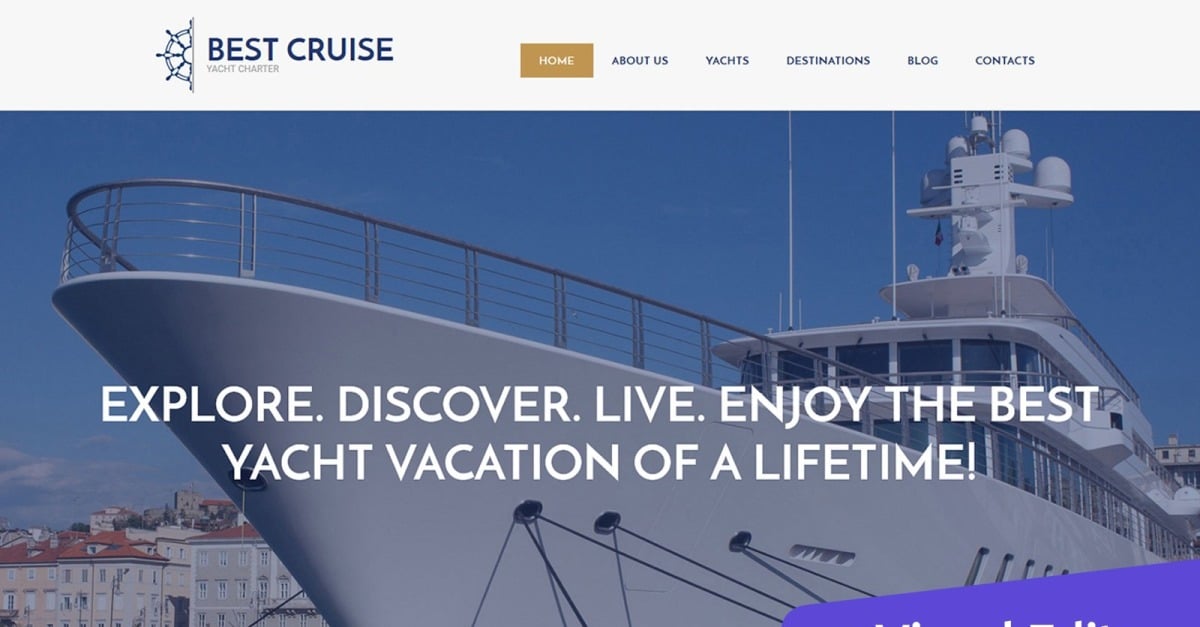In this screenshot from the "Best Cruise Yacht Charter" website, the top menu is displayed against a light blue background. On the left side, the company name "BEST CRUISE" is prominently featured in capitalized, blue font. Beneath it, in a much smaller grey font, the words "Yacht Charter" are written. To the left of the company name, the logo is depicted as the upper half of a ship's steering wheel, drawn in blue.

To the right of the logo, the menu items are listed. The currently selected menu item, "Home," is highlighted with a gold background and white font. The other menu items—"About Us," "Yachts," "Destinations," "Blog," and "Contacts"—are displayed in blue font against the light blue background.

Below the menu, a large photograph dominates the screen, presumably showing the bow of a yacht under a stunning blue sky. Overlaying the photo in white text are the words: "Explore, Discover, Live, Enjoy the Best Yacht Vacation of a Lifetime!"